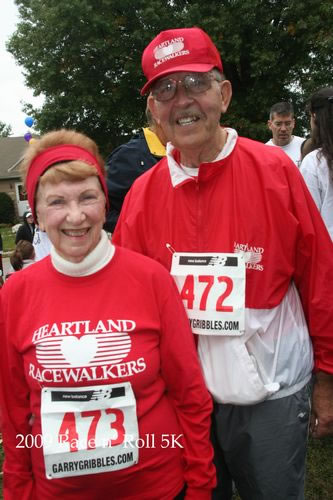In this image, an elderly couple is posing for a photo at what appears to be a marathon or a race event, as indicated by their number tags. The scene is set outdoors in a suburban neighborhood, visible from the large tree in the upper right corner and a bit of sky and house roof in the upper left corner. The woman, positioned on the left, has reddish hair pulled back with a red headband. She wears a long-sleeve red shirt with the text "Heartland Racewalkers" and a white heart graphic in capital letters, over a white turtleneck. Her race number, 473, is on a white tag with red numbers, along with the text "GaryGribbles.com" and part of "Roll 5k." Next to her, the man is dressed in a red and white rain jacket featuring the same logo and has the number 472 on his tag. He also wears a red hat and glasses. Both are smiling warmly at the camera, embodying a spirit of camaraderie and enthusiasm. Surrounding them, there is a small bush, a yard, and a group of people gathered in the background, adding to the lively and communal atmosphere of the event.